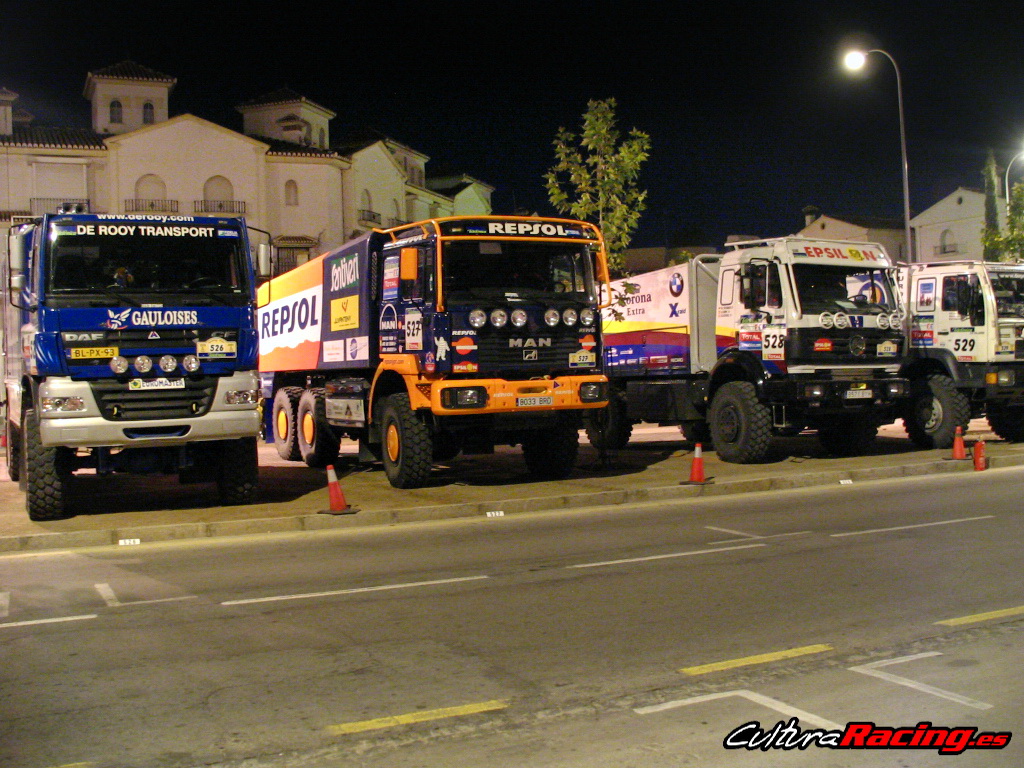This nighttime photograph features four large heavy-duty transport trucks lined up side-by-side off the side of a road, marked with the text "CulturaRacing.es" at the bottom right in red letters. The blue-purple truck on the left displays "DeRuey Transport" in white text. To its right, an orange-yellow truck bears the branding "Repsol" and "MAN." The two trucks on the far right are predominantly white with blue, red, and yellow stripes, featuring the names "Epsilon" and "CulturaRacing.es." Each truck is equipped with large tires, bright spotlights, and sporting different sponsor logos and numbers like 527, 528, and 529. The trucks are positioned behind a roadway marked with horizontal white and yellow lines and are flanked by orange traffic cones. In the background, under a dark blue-black sky, stands a large apartment building with cream or yellow trim, balconies, and illuminated by streetlights. A single tree highlights the center of the image, lit from below by a streetlight, contributing to the urban night setting.